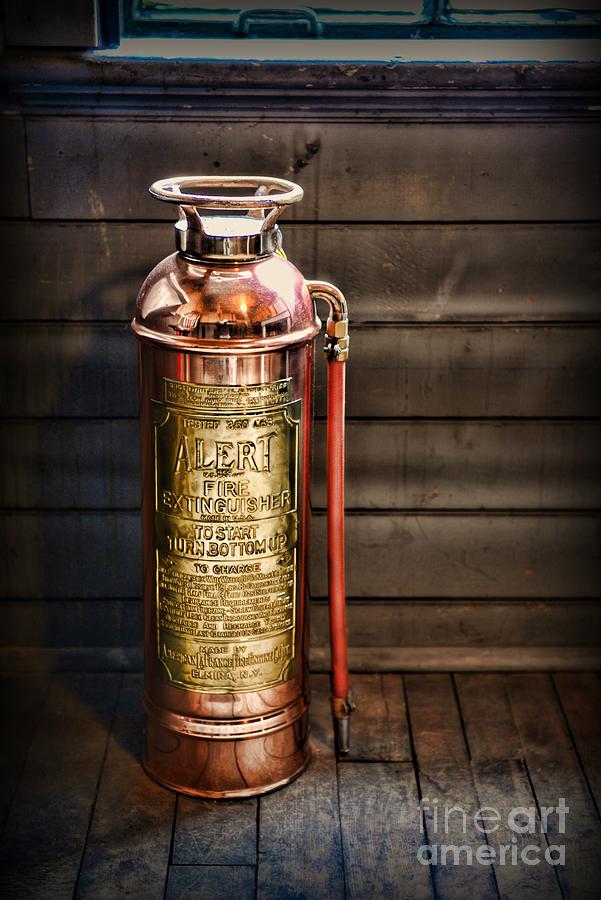The image features a vintage-style fire extinguisher positioned slightly left of center. The extinguisher has a distinctive round disc top with a large opening, transitioning into a dome-shaped, reflective, bronze-colored body. Its metallic surface gleams in coppery tones, complemented by a prominent golden label on the front. Although some words on the label are legible—such as "ALERT," "FIRE EXTINGUISHER," and "TO START, TURN BOTTOM UP"—the majority of the text is too small to read clearly. A gold or bronze nozzle extends to the right, bending downward to a long red hose that nearly touches the wooden floor. The hose terminates in a nozzle resting on the dark brown wood planks, which show signs of wear with light and dark stains. The backdrop consists of a wooden wall with horizontal planks, a window partially visible at the top of the frame, and the faint gray watermark "Fine Art America" in the bottom right corner.